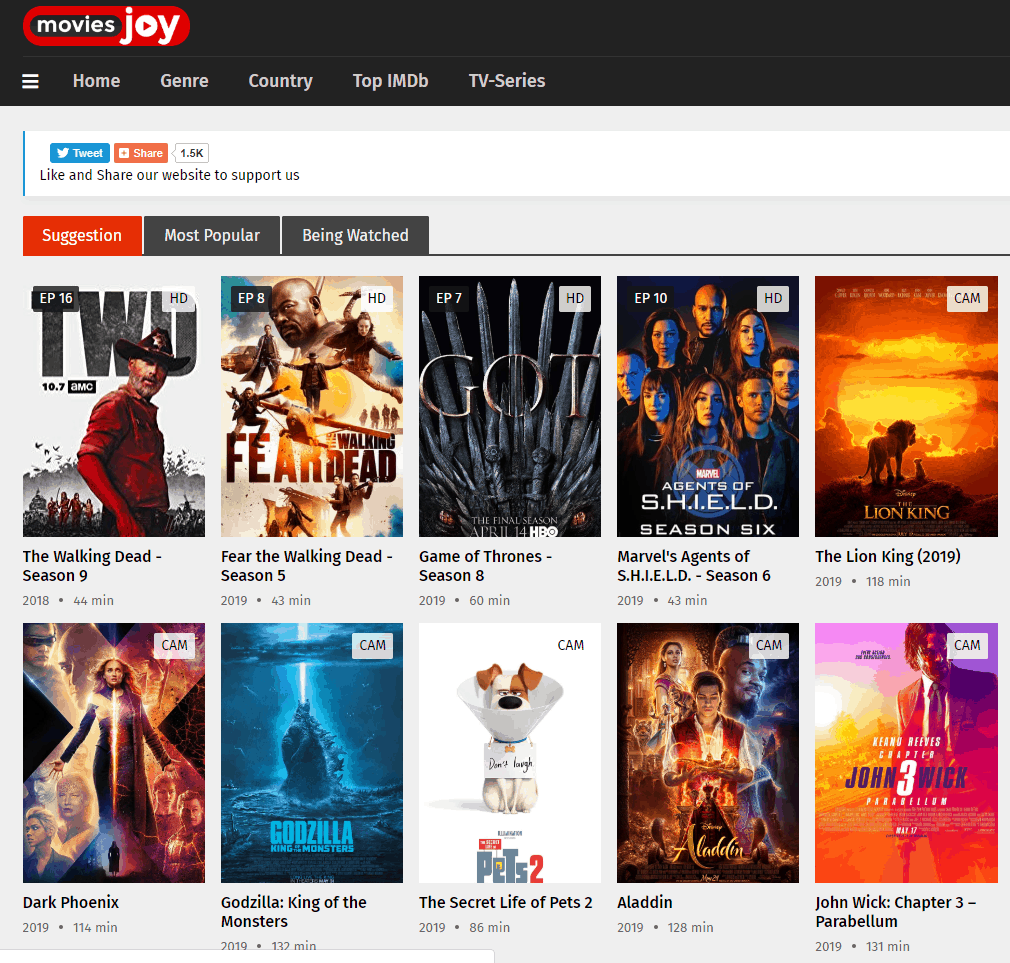This is a screenshot from a website dedicated to movies and TV series. At the top, there's a black navigation bar featuring a small red oval and the site name 'Movies Joy.' 'Movies' is displayed in a white font inside a black oval, while 'Joy' is in large white font with the 'O' styled as a play button. 

Below the main title, there is a menu with options: 'Home,' 'Genre,' 'Country,' 'Top IMDB,' and 'MTV Series,' all in white font. The webpage background is a soft gray. At the top, there's a white banner with black text urging users to "Like and Share our website to support us." Above this banner are social media buttons: a blue 'Tweet' button with a white Twitter icon and a green 'Share' button indicating '1.5K' shares.

Beneath the banner is another menu bar with 'Suggestion' highlighted in red, and 'Most Popular' and 'Being Watched' in black font. Below this, there are two rows, each containing five movie thumbnails. Each thumbnail displays the movie's cover art, title, running time, and release year. For example, the first thumbnail is for 'The Walking Dead: Season 9,' which was released in 2018 and has a running time of 44 minutes.